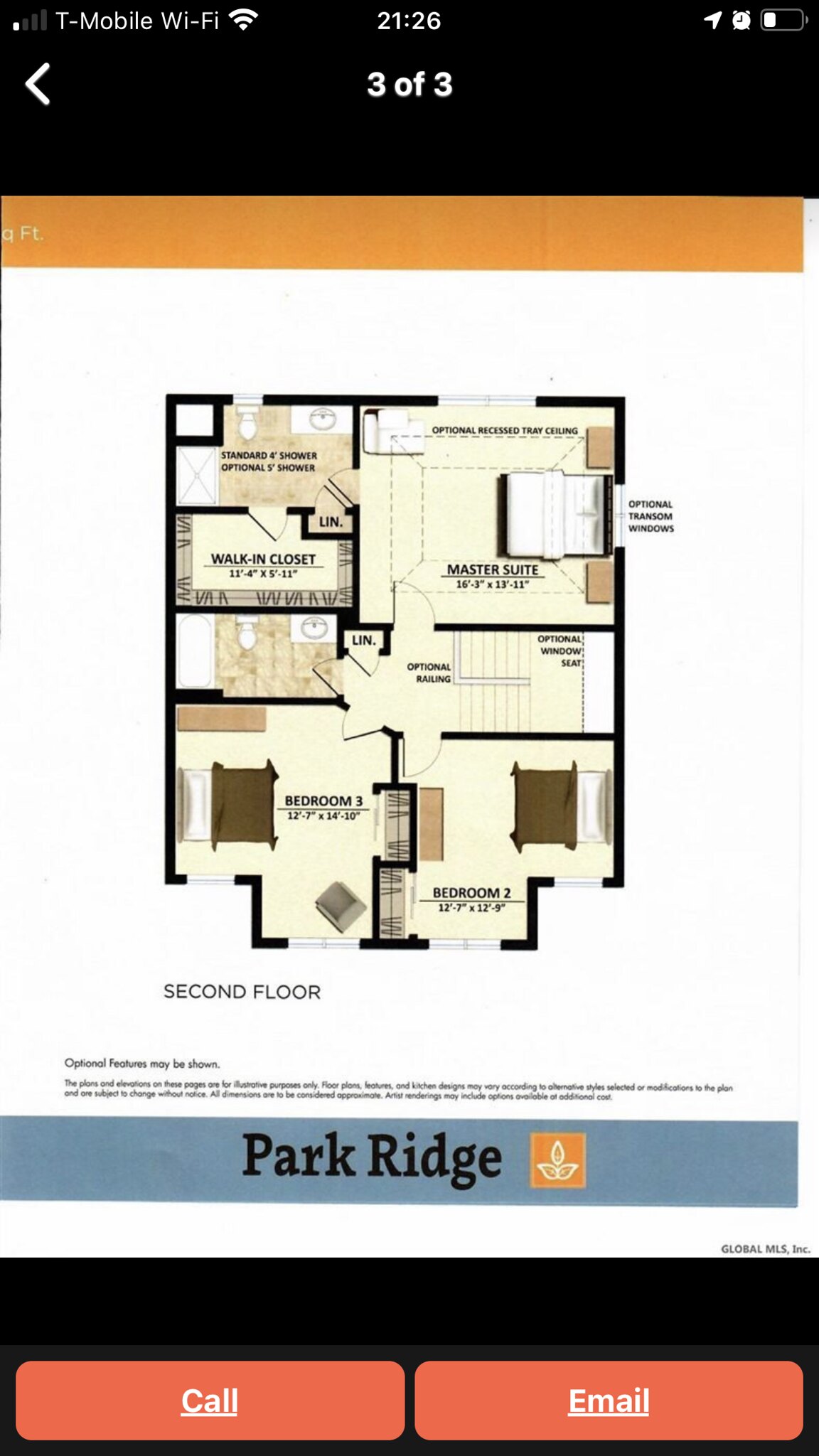**Detailed Caption:**

The image in portrait orientation is a cell phone screenshot. In the top-right corner, there is a single dot indicating the mobile network signal, followed by "T-Mobile Wi-Fi" and three signal bars fully lit up. The time displayed is 21:26. Adjacent to this, there is a white arrow pointing right, a clock icon showing nine o'clock, and a battery icon less than half full.

Below this status bar, a thick black strip spans the screen width, containing a left-pointing white arrow and centered text reading "3 of 3." 

Occupying the main section of the screenshot is a detailed floor map of a Park Ridge apartment's second floor. The diagram starts with an orange strip at the top, followed by a black outline of different rooms. 

**Key Details:**
- **Top left corner**: Indication of a standard four-foot shower with an optional five-foot shower.
- **Directly below it**: A walk-in closet measuring 11 feet 4 inches by 5 feet 11 inches.
- **Top right corner**: Features optional recessed tray ceiling and optional transom windows.
- **Master Suite**: Dimensions are 16 feet by 13 inches by 13 feet by 11 inches, located centrally on the diagram.
- **Bathroom**: Visible toilet and bathtub with optional railing and optional window seat indicated to the right.
- **Lower left of the diagram**: Bedroom three measuring 12 feet 7 inches by 14 feet 10 inches; outlines of beds are visible.
- **Right of this area**: Bedroom two measuring 12 feet 7 inches by 12 feet 9 inches with bed outlines.

Below the diagram, there is text indicating the second floor and a disclaimer regarding optional features, plan variations, and the approximate nature of dimensions. It states that the plans and elevations are illustrative, with potential modifications and additional costs for certain options.

A thick gray strip underneath the disclaimer reads "Park Ridge" and includes an orange logo with a yellow flower. Below this logo, the text "Global MLS, Inc." is present. Finally, at the bottom of the screenshot, a large black rectangle houses two oval buttons: a red "Call" button and an adjacent "Email" button.